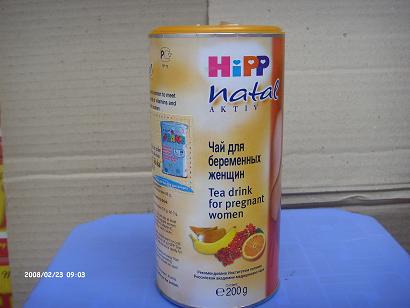This close-up photograph features a canister containing a specialized tea product for pregnant women. The canister prominently sits on a blue surface, with a plain white cardboard background enhancing its details. The canister is adorned with a paper label and topped with a bright orange lid that fits snugly into the opening. The label is bilingual, displaying text in both Russian and English. The company's logo, "HIPP," is vividly presented in colorful letters. The label showcases an assortment of fruit illustrations, including a whole orange, a half-cut orange, a banana, and some red berries. The overall labeling is primarily in a light orange hue, making the product visually appealing and informative.